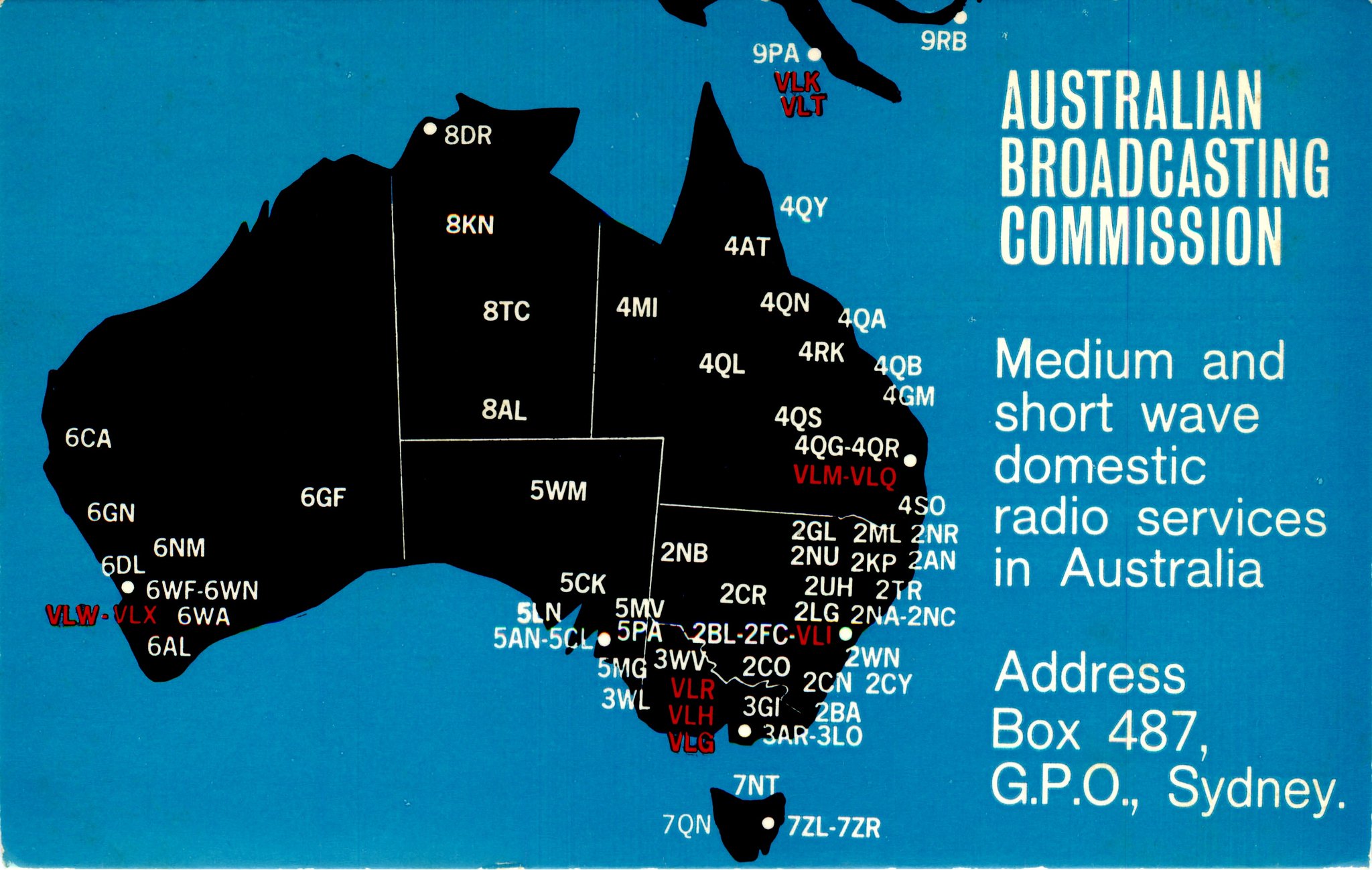This color image features a detailed map of Australia with a focus on its radio broadcasting services. Rendered in black against a blue background, the map is accentuated with white text. The top right corner of the image displays the title "Australian Broadcasting Commission," followed by the subtitle "Medium and Short Wave Domestic Radio Services in Australia" along with the address "Box 487 GPO Sydney."

The map of Australia is divided into six unspecified sections without explicit labels. Each section contains a series of three-character designations that are not defined within the image. For instance, the west coast features labels such as "6CA," "6GN," and "6NM," while the east coast includes designations like "2NR" and "2AN." These labels likely correspond to various radio stations or signal types.